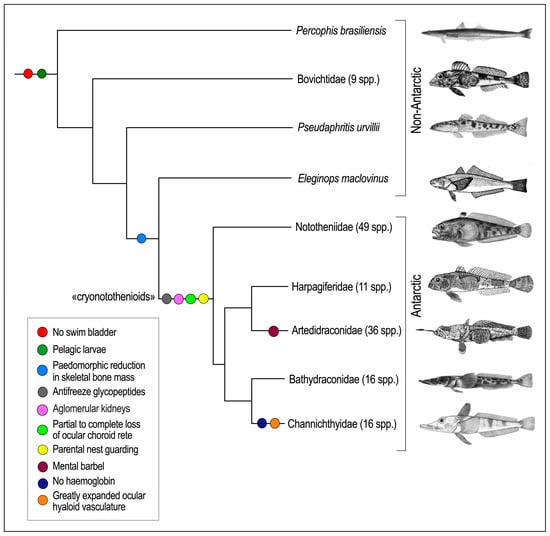The image is a detailed, square-shaped science chart with a thin black border. Dominating the right side of the chart are black-and-white illustrations of various fish species, organized into two groups: non-Antarctic fish at the top and Antarctic fish at the bottom. The non-Antarctic fish are generally long and thin, including recognizable species like a pike and a barracuda. Antarctic fish, in contrast, appear broader and more ominous. Each fish is annotated with its Latin name stacked to the left of the illustrations. 

Centered in the diagram, a flowchart extends from top to bottom, illustrating the genealogical relationships between the fish species. To the left, mid-way down the image, there's a legend, marked by colored circles (red, green, blue, gray, pink, and green) each representing specific biological features like "no swim bladder" and "mental barbel." This legend provides detailed information about the anatomical and physiological characteristics of the fish, linking back to the colored dots next to each fish in the flowchart. At the bottom left, a gray rectangular box further categorizes additional information present in the chart. This combination of fish illustrations, Latin names, a detailed legend, and an informative flowchart makes the chart a comprehensive guide to understanding the species' distinguishing features and their evolutionary relationships.